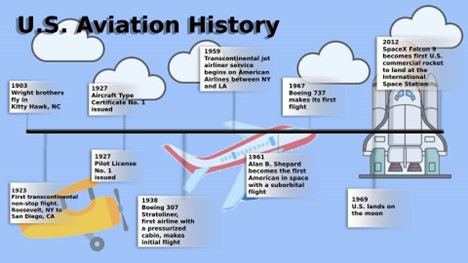The image is a small rectangular poster, approximately three inches wide and two inches high, titled "U.S. Aviation History" in bold black print on a light periwinkle blue background in the upper left-hand corner. A solid black horizontal line runs across the poster, serving as a timeline with lines extending vertically above and below it. The poster features ten distinct blocks of text, each inside a gray box that fades as it moves to the right. Each block marks a significant event in U.S. aviation history, beginning with the Wright Brothers' first flight in Kitty Hawk, North Carolina in 1903, and culminating in SpaceX's Falcon 9 becoming the first U.S. commercial rocket to dock at the International Space Station in 2012. The background includes five clouds and illustrations of various aircraft, including two airplanes and a spaceship. Key milestones highlighted include the first transcontinental nonstop flight in 1923, the issuance of Aircraft Type Certificate Number 1 and Pilot License Number 1 in 1927, the inaugural flight of the pressurized Boeing 307 in 1938, the start of transcontinental jet airliner service by American Airlines in 1959, Alan Shepard's 1961 suborbital flight as the first American in space, the 1947 first flight of the Boeing 737, and the U.S. moon landing in 1969.